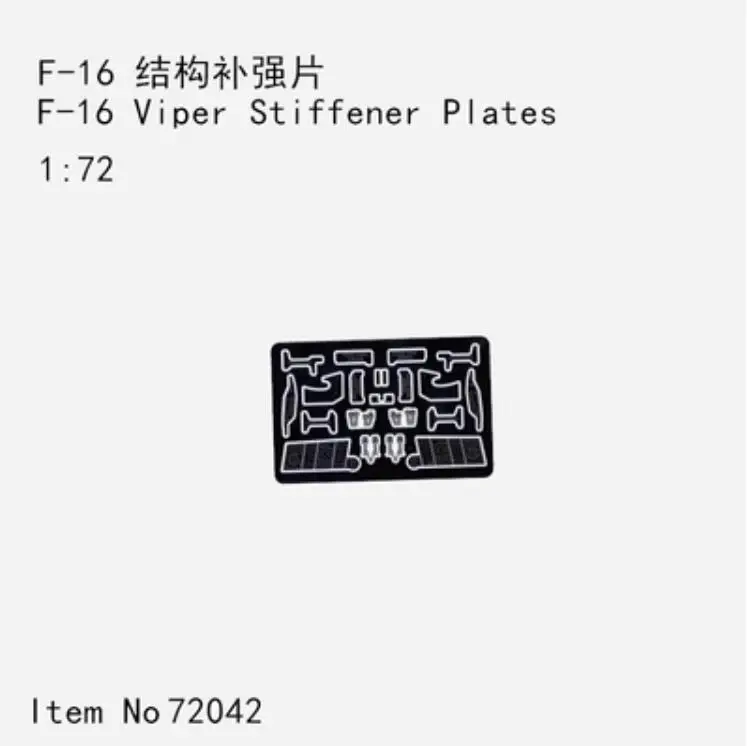The image showcases a central black rectangle against a gray background, resembling parts for a model airplane, specifically labeled as "F-16 Viper Stiffener Plates." The black object features intricate, irregularly shaped white outline symbols that mirror each other along the center, creating the appearance of parts cut out from a larger frame. The text at the top reads "F-16" followed by what appears to be Chinese or Asian kanji characters, then "F-16 Viper Stiffener Plates." Directly below this text, the scale is indicated as "1:72." Additionally, "Item number 72042" is noted in black text in the bottom left corner. The overall presentation suggests it is a detailed component meant for model airplane enthusiasts, possibly featured on a product listing for an online store.